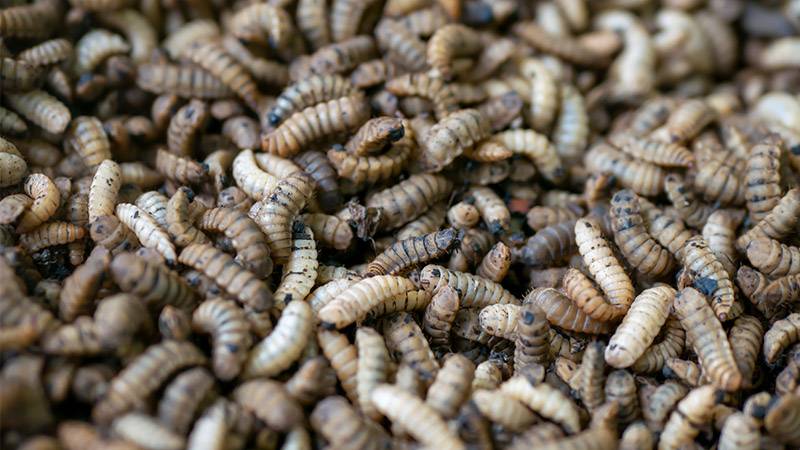This image is a detailed close-up photograph of a massive swarm of worms, possibly maggots or grubs, filling the entire frame. The worms are predominantly light brown, though their coloration varies from whitish and beige to darker brown. Their segmented bodies are visible, with around a dozen joints each, giving them a distinctly wriggling appearance. Many of them bear small black dots on their backs, and some have visible eyes, particularly those in the image's center. The worms appear to be dirty, as if they have been burrowing through soil. The scene is densely packed, with easily hundreds of these creatures, creating a sense of uncountable numbers. The image has a focused central area, making the eyes and heads of the central worms more defined, while the worms towards the edges, especially in the bottom left corner, appear blurrier and less distinct. There is nothing else in the photograph, just a top-down view of this swarming mass of worms.